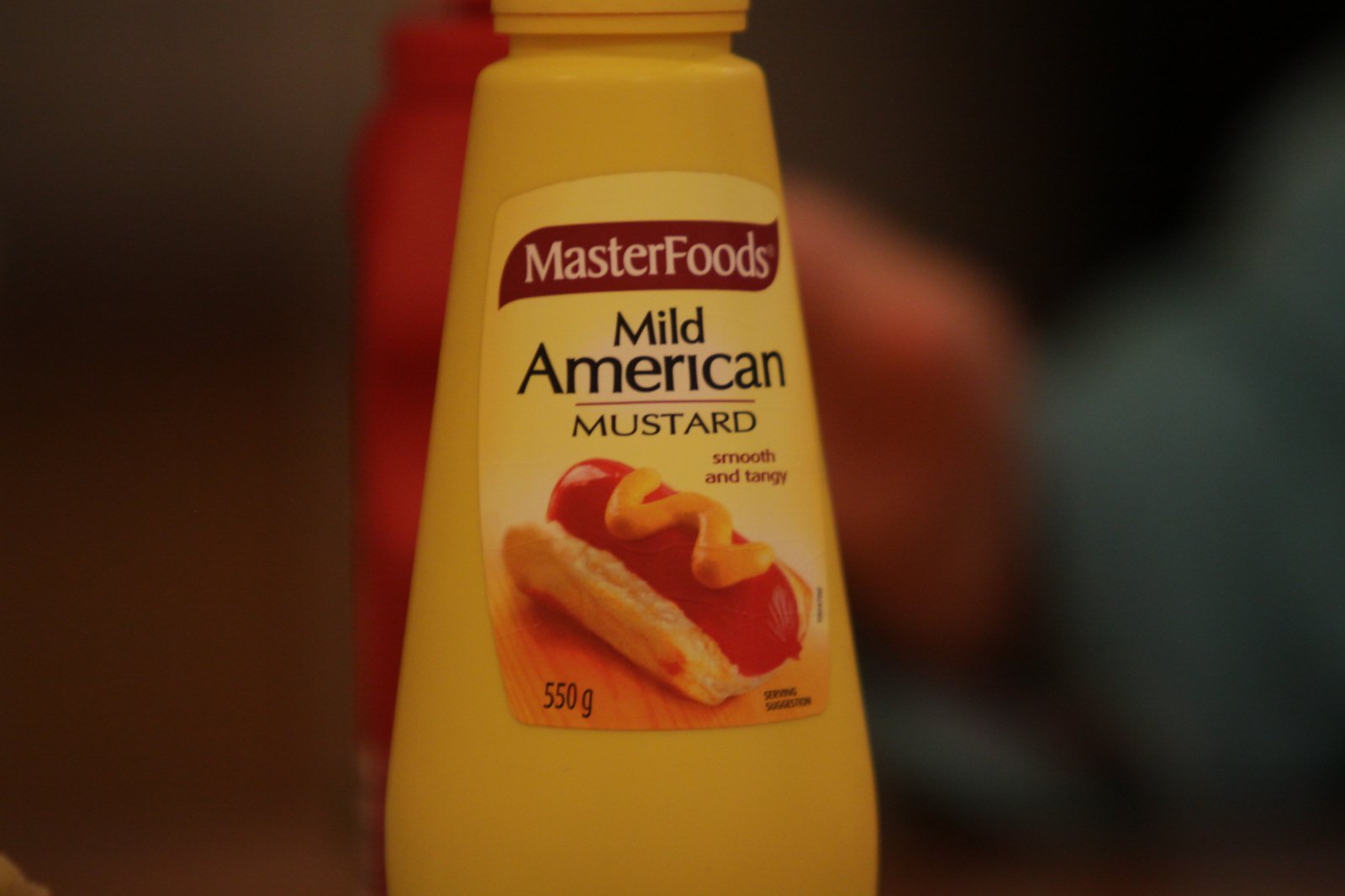This image showcases a classic yellow plastic bottle of mustard standing upright, captured from a side view, with its bottom out of frame. The bottle has a cylindrical shape that tapers slightly upward. Its label features a red banner at the top with "Master Foods" written in white letters. Below, in black letters on a yellow background, it reads "Mild American Mustard." A central image displays a hot dog in a bun with a bright yellow, zigzag line of mustard on top. Additional text on the label includes "Smooth and Tangy" and "550 G." The background is blurred, showing indistinct shapes and colors, including a silhouette of fingers that seem to be holding the mustard bottle and hints of brown, black, blue, and red elements. The overall focus is sharply on the mustard bottle, emphasizing its traditional color and design.